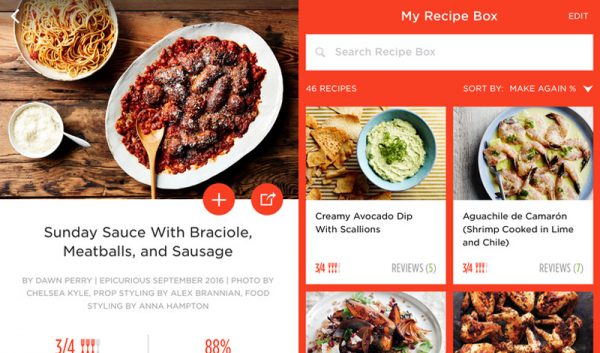The image showcases a detailed screenshot of a website, divided into two sections:

On the left-hand side, there is a vibrant photograph that captures a delectable spread of Italian cuisine. The centerpiece is a white bowl filled with spaghetti noodles generously topped with a rich red sauce. Adjacent to this, a large white platter holds numerous meatballs, also drenched in red sauce. Completing the setting is a wooden spoon placed on the rustic, medium-brown wooden table, which adds a charming, homely touch. Additionally, a small white bowl, presumably containing Parmesan cheese, sits nearby. 

Below the photograph, a white box with black text reads: "Sunday Sauce of Braccioli Meatballs and Sausage by Don Perry, Epicureus, September 2016. Photo by Chelsea Kyle, Prop Styling by Alex Branny, and Food Styling by Anna Hampton." It also mentions that the recipe has received a rating of three out of four forks and an overall 88% rating.

On the right-hand side of the screenshot, there's a red sidebar labeled "My Recipe Box." At the top of this sidebar, there's a search bar captioned "Search Recipe Box." The sidebar indicates that there are 46 recipes saved. At the top of the list, the first two images are featured: a "Creamy Avocado Dip with Scallions," which shows a blue bowl filled with a green dip and accompanied by various chips, and "Aguachile de Camarón (Shrimp Cooked in Lime and Chili)," displayed on a blue plate with shrimp in a vibrant green sauce.

The entire scene conveys an intimate yet inviting culinary experience, meticulously styled and photographed, capturing both the essence of home-cooked comfort and the precision of gourmet detail.